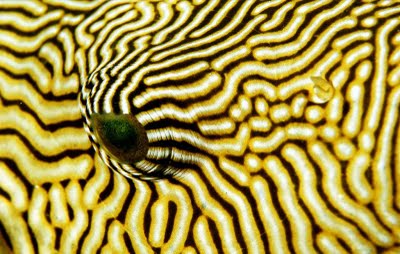This image depicts a highly detailed, close-up view of an unknown organism's eye, captured through what appears to be a microscope. Dominating the image are striking yellow and black stripes, with the yellow sections slightly thicker and outlined in a darker shade of yellow. These stripes traverse the field of view, occasionally appearing broken and pieced together, but consistently forming a segmented pattern. In the center of this intricate tapestry, a peak rises toward the camera, adorned with the same yellow, black, and occasional white stripes. At the tip of this cone-like structure is a green dot, which constitutes part of the bulging eye, surrounded by a faint brown border. The eye itself is mesmerizing, with its greenish-brown hue adding a layer of mystery and beauty to the organism, whose body remains out of view. Collectively, the elaborate pattern and vibrant colors evoke a sense of both spookiness and fascination, hinting at the eye possibly belonging to a snake, frog, or another amphibian.